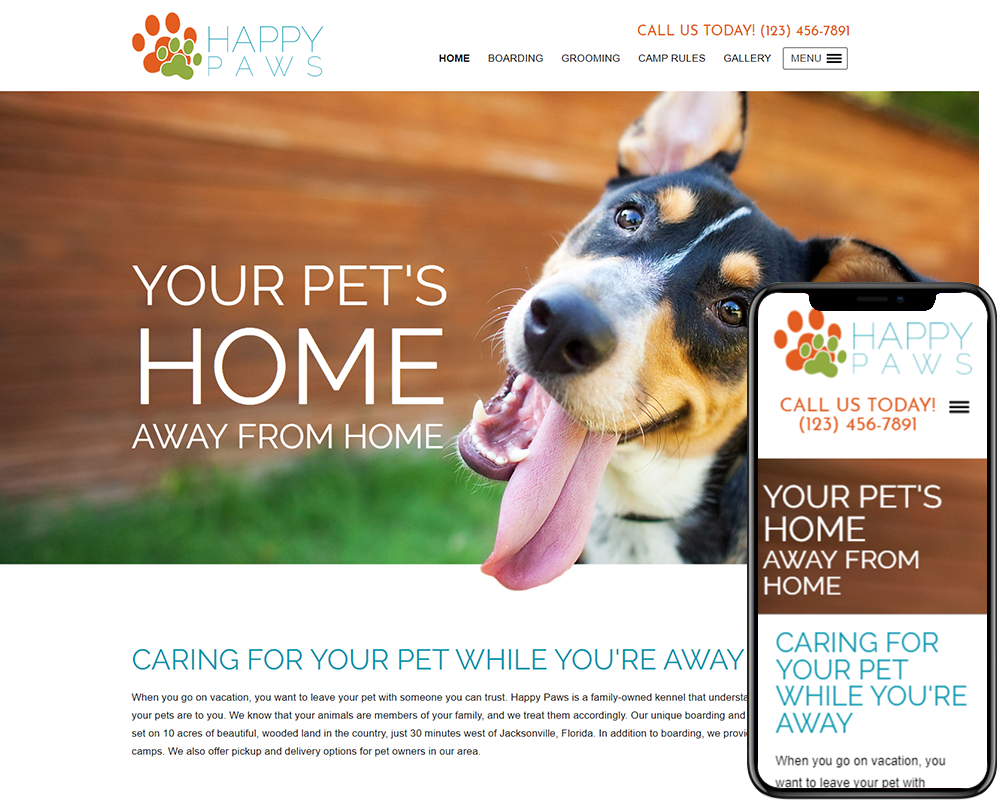**Detailed Caption:**

This advertisement showcases the "Happy Paws" website, featuring their vibrant and visually appealing design. The top of the page includes the Happy Paws logo comprised of two paw prints—a large orange one and a smaller olive-green one. The brand name "HAPPY PAWS" is displayed prominently in a captivating blue, all-uppercase text. The spacing between the letters of "HAPPY" and particularly "PAWS" is noticeably generous, adding a modern touch to the title. 

In striking orange, all-capital letters below the logo, the website urges visitors to "CALL US TODAY," followed by the contact number: "123-456-7891".

Directly beneath the contact information, the site’s navigation menu is visible, including options such as Home, Boarding, Grooming, Camp Rules, Gallery, and a dropdown menu box. Currently, the Home page is selected, emphasizing the slogan "Your pets' home away from home" in bold, white, capitalized text.

A standout feature on this page is a picture of a tan, black, and white dog with a highly realistic tongue hanging out. The tongue’s 3D appearance makes it seem as though it is popping out of the screen, though it doesn't quite fit the dog's mouth, hinting it may be AI-generated. The dog's expressive face and detailed fur texture, particularly the black and white pattern around its nose and chest, exude friendliness and trustworthiness.

Further down, in large, blue, capitalized text, the site reassures pet owners with the message, "CARING FOR YOUR PET WHILE YOU'RE AWAY.” Below this, a brief description begins: "When you go on vacation, you want to leave your pet with someone you can trust. Happy Paws is a family-owned kennel that understands your pets'..." Unfortunately, the text is partially cut off by another overlapping section, but it emphasizes the kennel’s familial and trustworthy approach, hinting at their understanding of pets as beloved family members.

The informative text continues, partially covered, describing the setting: "Our unique boarding and block...set on 10 acres of beautiful wooded land in the country, just 30 minutes west of Jacksonville, Florida. In addition to boarding, we provide..." This section is incomplete but indicates additional services like camps and pet pickup and delivery within the area.

The lower part of the page features an image of a mobile phone displaying a miniature version of the Happy Paws website. It includes the same distinctive logo, phone number, and a simplified menu, reiterating, "Your pets' home away from home" and "Caring for your pet while you're away," ensuring a seamless and consistent user experience across devices.

Overall, this detailed and engaging depiction of the Happy Paws website illustrates its comprehensive pet care services, user-friendly design, and commitment to maintaining a home-like environment for pets.